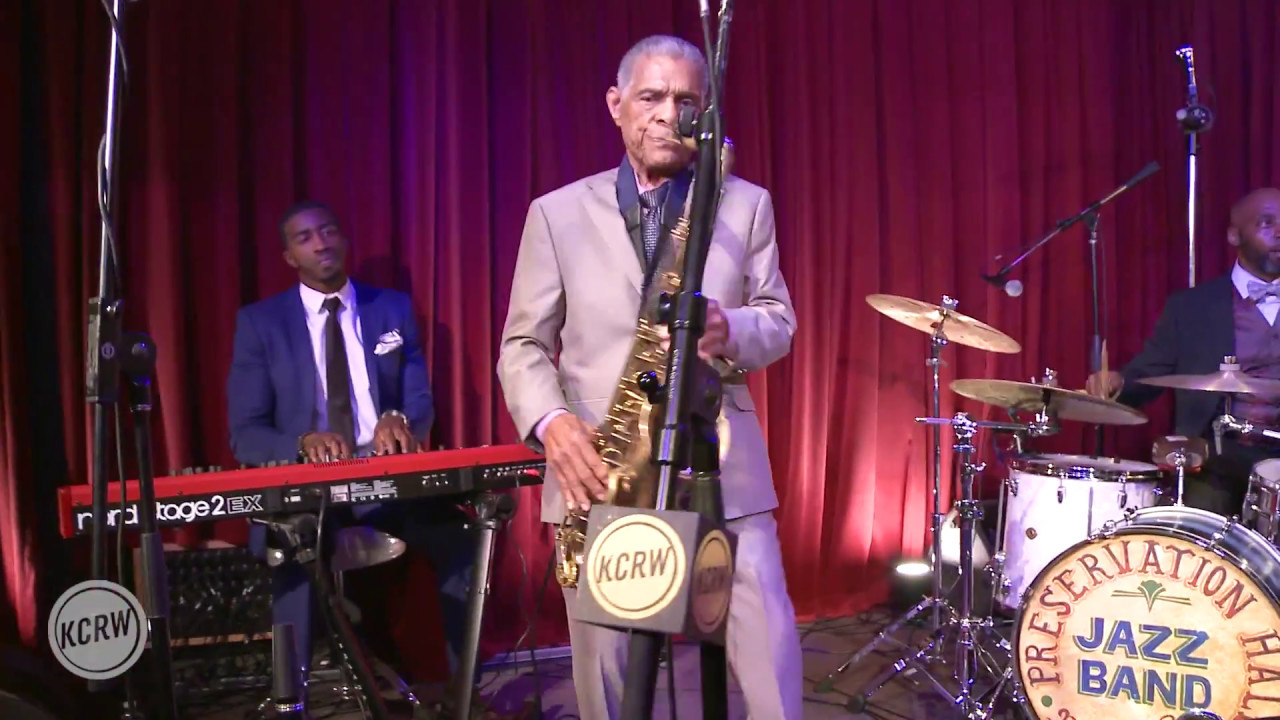The image showcases a performance by the Preservation Hall Jazz Band on a stage, likely during a television or talk show. The red curtain in the background is fully closed, emphasizing the musicians center stage. In the spotlight is a black man in a metallic gray suit adorned with a blue shirt and tie, engrossed in playing the saxophone. To his left, a black man in a blue suit, black tie, and white shirt sits at a red keyboard, his gaze focused on the saxophonist. On the right, another black man in a black suit, blue vest, and blue bow tie energetically plays the drums, with "Preservation Hall Jazz Band" prominently displayed on the drum set. The KCRW logo is visible both on the microphone in front of the saxophonist and at the bottom left corner of the screen, reinforcing the show's branding. The scene is rich with musical equipment, capturing the essence of a live, intimate jazz performance.